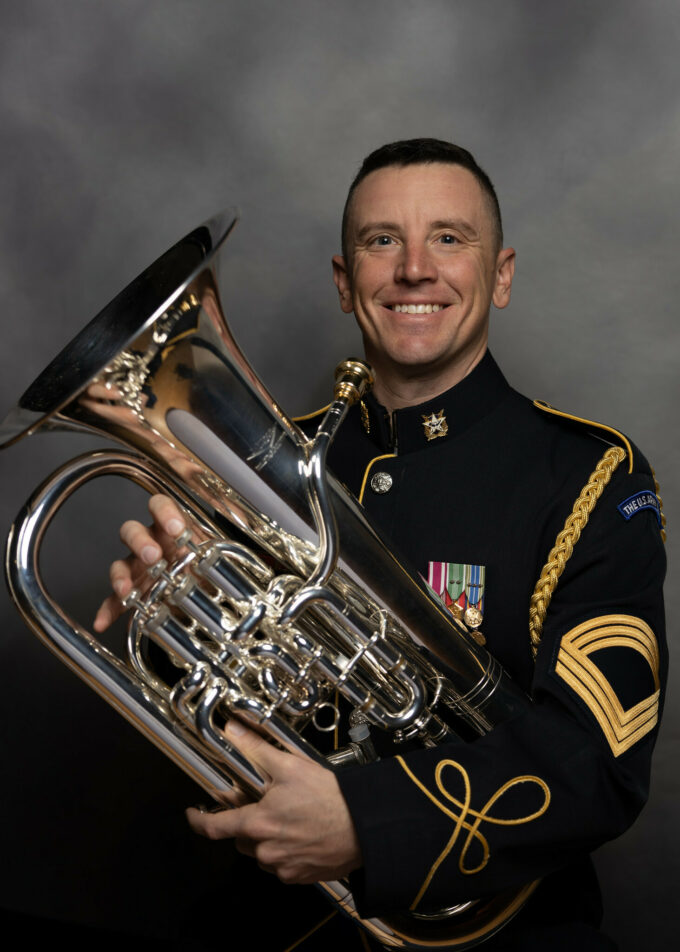This is a portrait of a man in a distinguished West Point-style dress uniform, characteristic of a military band member. The uniform, a dark blue with gold trim, features very high collars that extend partway up his neck. Adorning one of the neck flaps is a silver star-shaped insignia with a gold background, signifying his rank and achievements. On his left arm, there are sergeant stripes in yellow, consisting of three separated by dark lines, and a series of looping gold cords near the wrist which continue up the upper arm. His multiple badges and pins further emphasize his high rank. The man, who is smiling warmly and showcasing white teeth, has a short military-style haircut and brown eyes. He stands in front of a cloudy, grayish portrait background, which accentuates him as the bright focal point of the image. His prominent dimples and large ears add to his approachable demeanor. Holding a shiny silver tuba, with his fingers positioned on the valves, he clearly takes pride in his role as a band member, reflecting a deep sense of duty and honor.